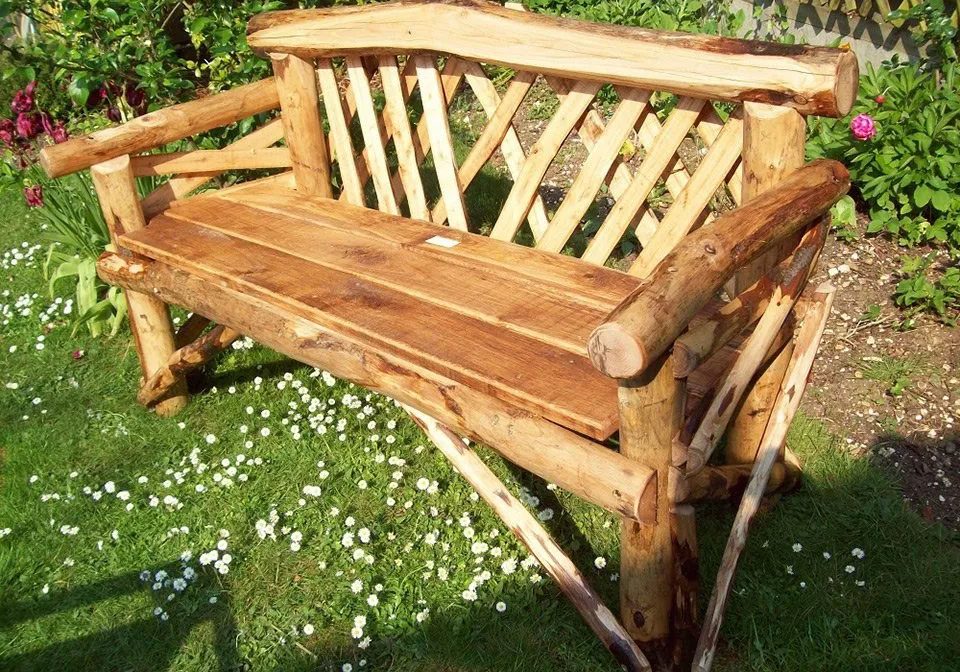This up-close photograph captures a rustic wooden bench nestled in a lush, green grassy area. Viewed from a slightly elevated angle, the bench is surrounded by a multitude of small, white flowering weeds scattered across the grass. The seating surface consists of three flat wooden planks, while the backrest features diagonally positioned slats of wood supported by logs at either end. The armrests and legs of the bench are crafted from small logs, and an additional log serves as a brace just beneath the front edge of the seat. Behind the bench, low green shrubs adorned with delicate purple flowers provide a picturesque backdrop, enhancing the serene, natural setting.